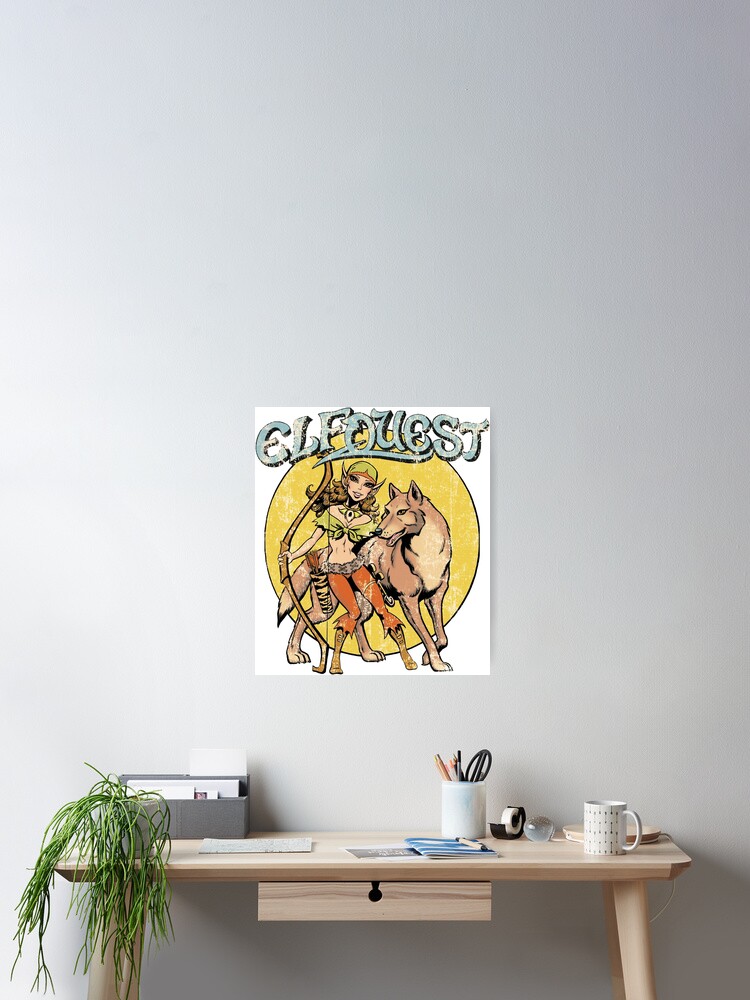The image depicts a minimalist, tan-colored wooden desk pushed up against a painted light, possibly lavender or grayish-white wall, with sunlight streaming into the room. The desk, which has a butcher block style and an unfinished appearance, measures approximately five feet in length and a foot and a half in width. It features a single central drawer about 16 inches long and 4 inches tall, adorned with a black knob handle. 

Atop the desk is a white spotlight lamp with two metal arms connected by a central hinge, allowing for adjustable lighting. There is a white coffee mug filled with pencils, pens, and scissors, and another white coffee mug sitting alone on the right corner. A plant is placed on the left side of the desk. 

In the background, there's an animated poster that reads "Clear Fest," with art that appears to depict characters from the "Elf Quest" series. A file cabinet is partially visible behind the plant, adding a touch of practicality to the home office setup.